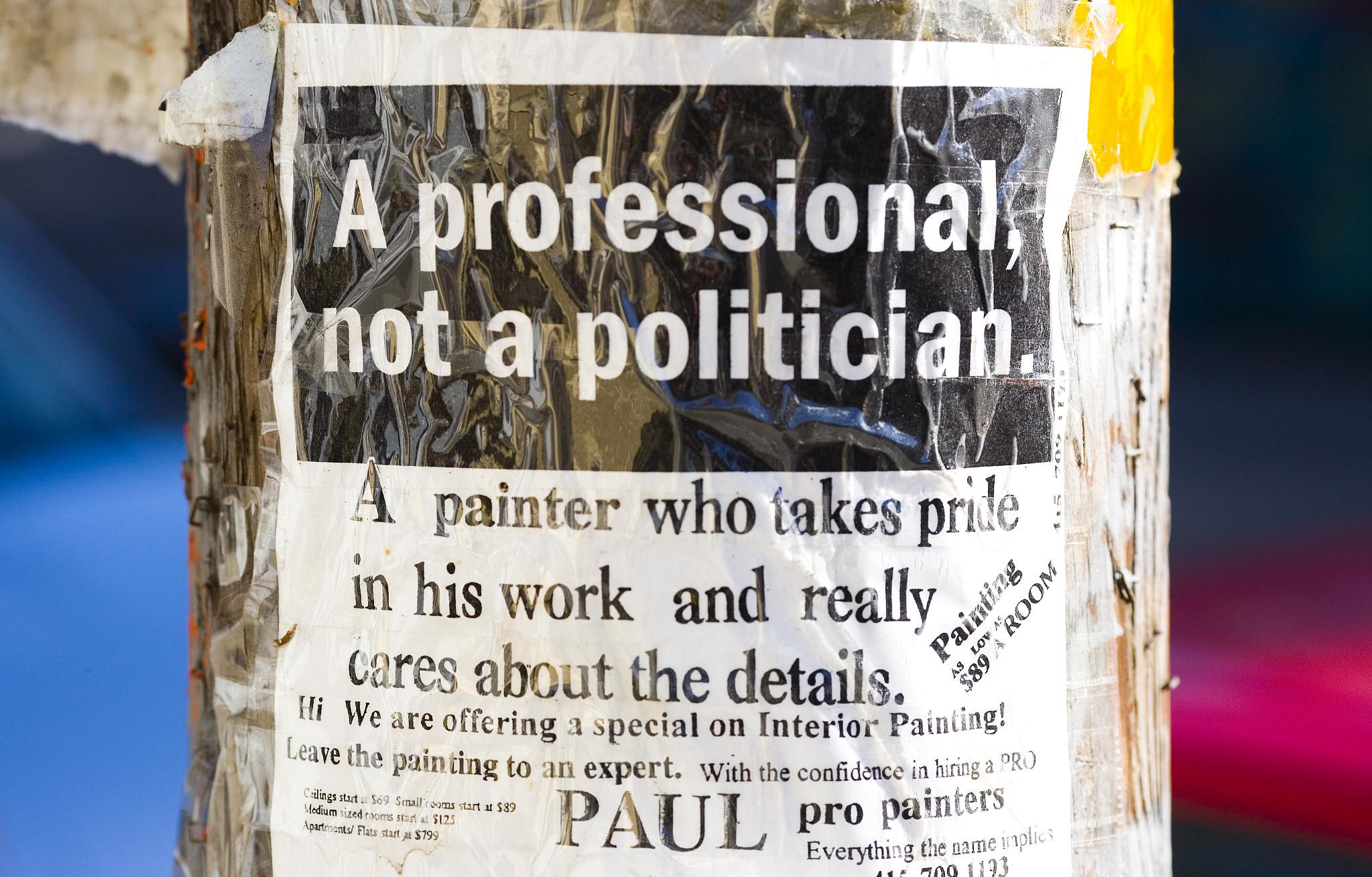This color photograph is a close-up of a worn, wooden lamppost covered with many old staples and layers of aged tape, along with a splash of random yellow paint. Affixed to this lamppost using clear tape is a partially visible bulletin promoting painting services. The top section of the bulletin features a black rectangle with white text that reads, "A professional, not a politician." This black rectangle is slightly askew, adding a casual, homemade touch to the flyer. Below, the bulletin transitions to a plain white paper with neat black print detailing the services offered. The text highlights a painter who prides himself on his meticulous work and attention to detail. It reads: "Hi, we are offering a special on interior painting!" Followed by "Leave the painting to an expert with the confidence in hiring a pro. Paul Pro Painters—everything the name implies." Although the phone number is cut off at the bottom, some very small, unreadable print can be seen in the bottom left corner, hinting at possibly more detailed contact information or disclaimers. The overall visual suggests a seasoned lamppost that has hosted numerous bulletins over time.